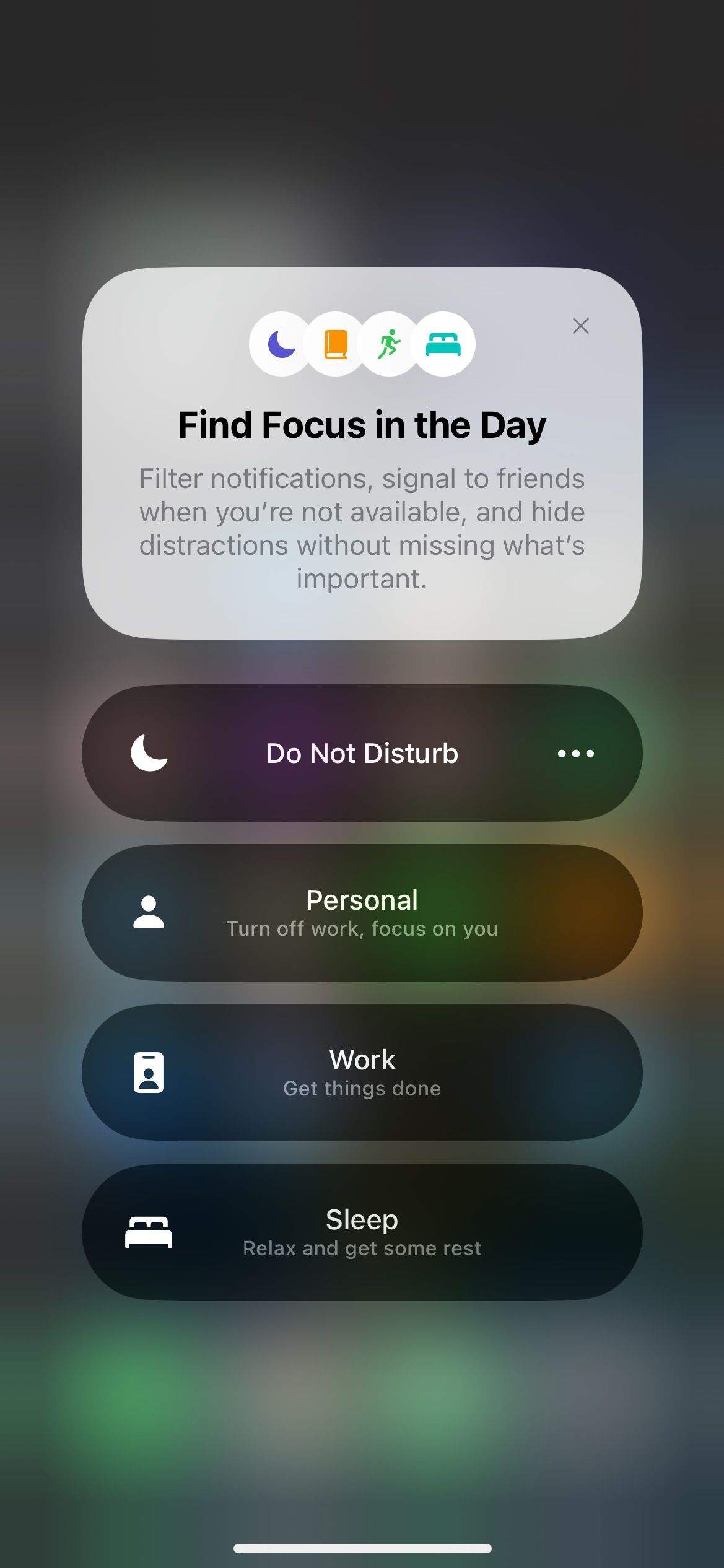The image appears to depict an interface resembling a meditation or mindfulness app, potentially also serving as a lock screen or control hub for a smartphone. The main window prominently displays the message "Find focus in the day," hinting at the app's purpose of enhancing concentration and reducing distractions. Below this main message, there are four subsidiary panels labeled "Do Not Disturb," "Personal," "Work," and "Sleep." Each panel is accompanied by respective icons, suggesting their distinct functionalities. The "Do Not Disturb" panel features a standard three-dot menu, indicating additional configuration options. Although the other panels lack these dots, it is unclear whether they are similarly configurable. The top container reiterates the message "Find focus in the day," reinforcing the app's focus-centric theme. It alludes to features like filtering notifications, signaling availability status to friends, and hiding distractions without missing crucial updates. The background consists of a semi-transparent overlay, lending an "appy" aesthetic to the interface.